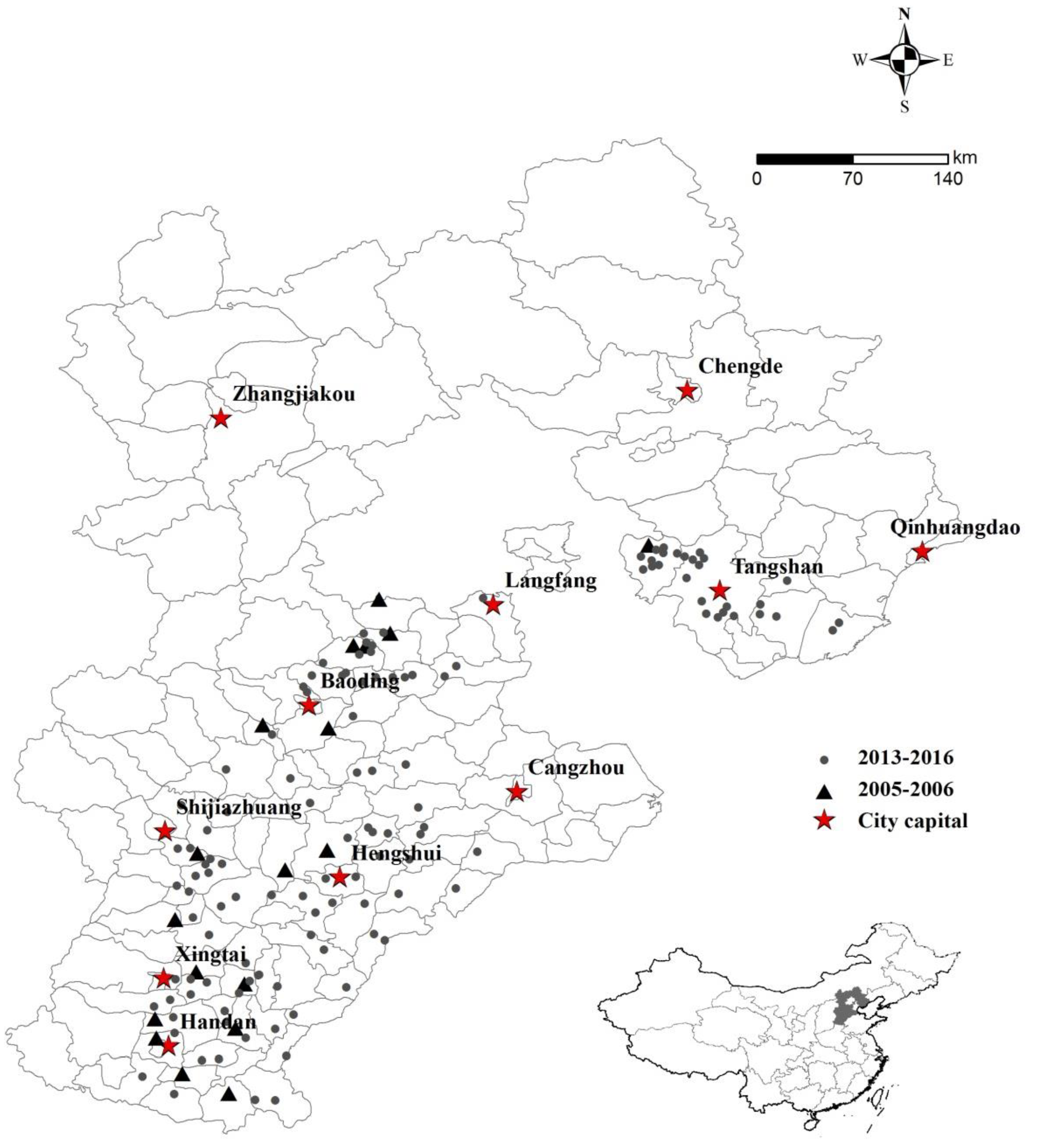The image is a detailed black-and-white map of China, highlighting various regions and their subdivisions, potentially equivalent to counties or states. Major cities like Hangzhou, Xingtai, and Tangshan are marked, with red stars indicating city capitals. The legend on the right explains the symbols: dots represent the years 2013 to 2016, triangles represent 2005 to 2006, and red stars mark city capitals. In the lower left, a smaller inset displays the entirety of China with the mapped region blacked out, while a compass in the top right indicates directions. The map also includes a kilometer scale, ranging from 0 to 140 kilometers, adding to its detailed informational content.